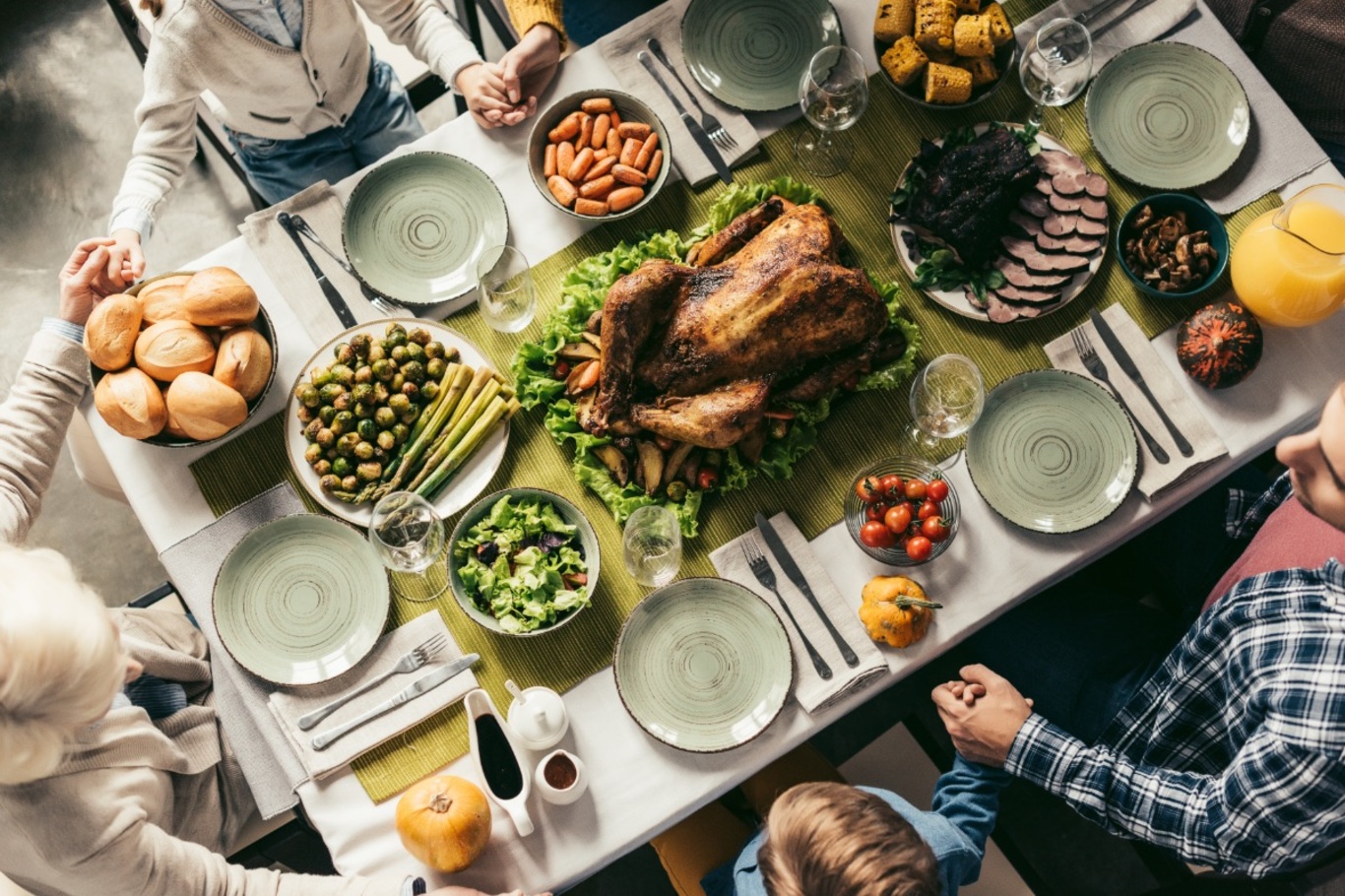This is an overhead photograph capturing a family gathered around a Thanksgiving table, hands held in a gesture of unity, likely sharing a moment of prayer. The rectangular table is adorned with a green fabric runner extending through its center. The table centerpiece features a browned whole turkey resting on a bed of lettuce. To the right of the turkey is a large white plate with sliced ham and greens, while to the left, there is a plate of Brussels sprouts and asparagus. The lower part of the table has a small bowl filled with lettuce, and beside it, a glass jug of orange juice. There are numerous wine glasses scattered around the table, all empty. In the top left corner, a bowl of bread rolls stands next to a bowl of baby carrots. In the top right, there is a bowl filled with corn cobs. Additional details include some pumpkins and potentially other vegetables like tomatoes and potatoes. Each place setting features an empty ceramic white plate, accompanied by a napkin with a fork and knife placed on it. The table is set for six individuals, including an older woman with white hair and a child holding a man's hand, who is wearing a red shirt and plaid flannel. The scene has a warm and staged feel, capturing the essence of a traditional family gathering.